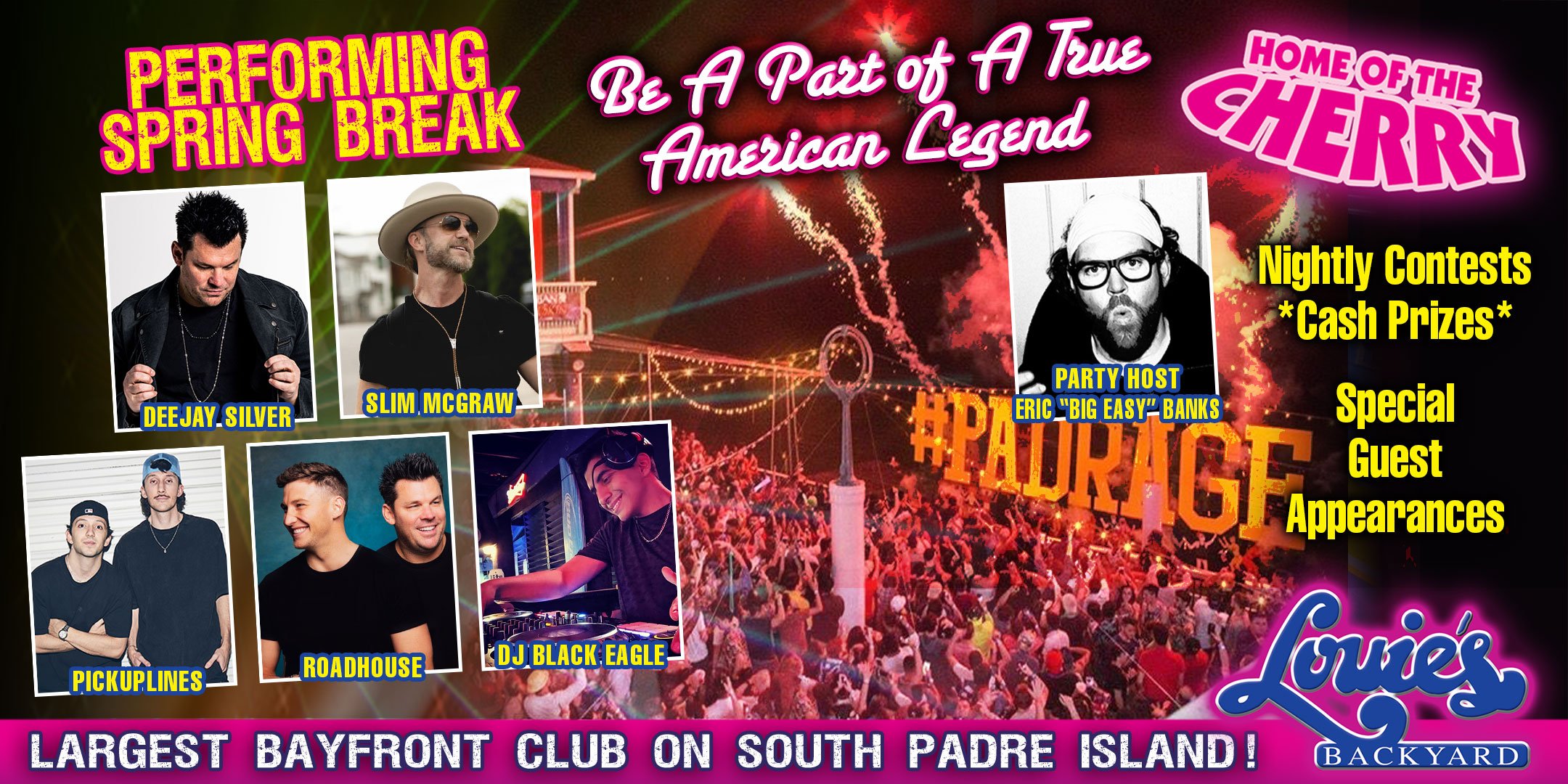This promotional poster for a nightclub event features a vibrant background with a crowd enjoying a lively event. On the left side, five photographs of musicians are displayed, showcasing DJ Silver, Slim McGraw, Pickup Lines, Roadhouse, and DJ Black Eagle. At the top left corner, the text "Performing Spring Break" is prominently written in yellow. The middle of the poster features the phrase "Be a Part of a True American Legend" in bold pink and white letters. On the right side, a photograph of the party host, Eric "Big Easy" Banks, is shown with accompanying text beneath it reading "Party Host, Eric, Big Easy Banks." Adjacent to this picture are details in yellow text that highlight additional features of the event, including "Home of the Cherry, Nightly Contests, Cash Prizes, Special Guest Appearances." At the bottom of the poster, a pink horizontal strip states "Largest Bayfront Club on South Padre Island" in white text. Finally, in the bottom right corner, the club's name "Louie's Backyard" is displayed in blue, italicized text, with "Backyard" in a serif Times New Roman font beneath it.